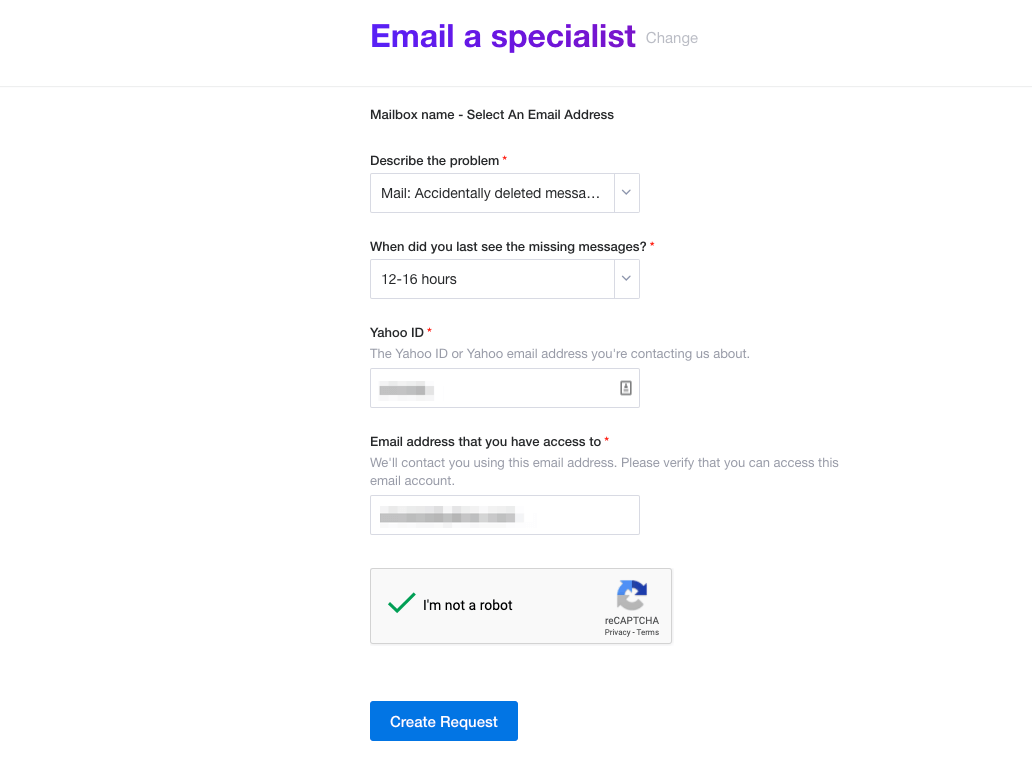This image details the process of an email specialist changing a mailbox name and selecting an email address to describe a problem involving accidentally deleted messages. The user is prompted with a question, "When did you last see the missing messages?", where a response of "12-16 hours" is filled in. The field requests for the Yahoo ID, or Yahoo email address you are contacting about, along with an additional email address that is accessible. There is a verification prompt to ensure access to the provided email account. At the bottom, there is a reCAPTCHA verification box labeled "I'm not a robot", which is checked, enabling the user to confirm their identity. Below this, a blue "Create Request" button is visible to submit the request. The image features a color palette comprising purple, black, white, green, and blue.